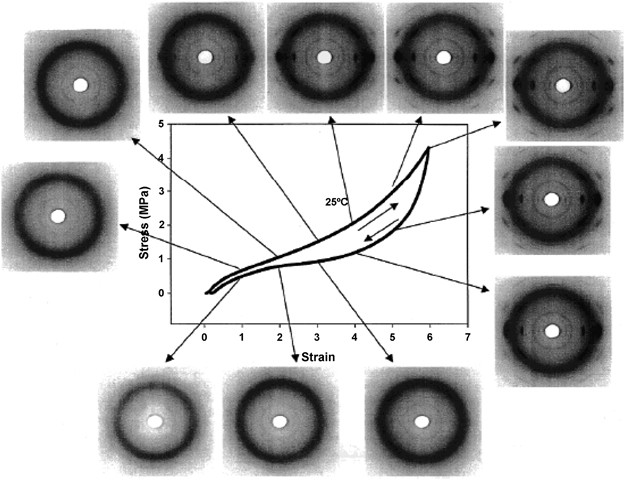The image is a detailed black and white stress-strain diagram, showcasing a graph with stress (MPa) on the vertical y-axis ranging from 0 to 5 and strain on the horizontal x-axis ranging from 0 to 7. The diagram features a primary curve that rises gently and another that curves downward, both starting from the same initial point and eventually converging. At the center of the graph is a label indicating the temperature, "25 degrees centigrade."

Surrounding the central graph are 11 small, black and white images, each featuring a circular shape with a black outer ring, a gray interior, and a bright white dot at the center. These images appear to represent various levels of stress and strain, with arrows from the central graph pointing to each one. The circles show varying degrees of distortion, thickness, and additional dots, resembling microscopic or x-ray images. These detailed visuals provide a representation of different material states under stress and strain conditions, but the specific meanings of these variations remain unclear.